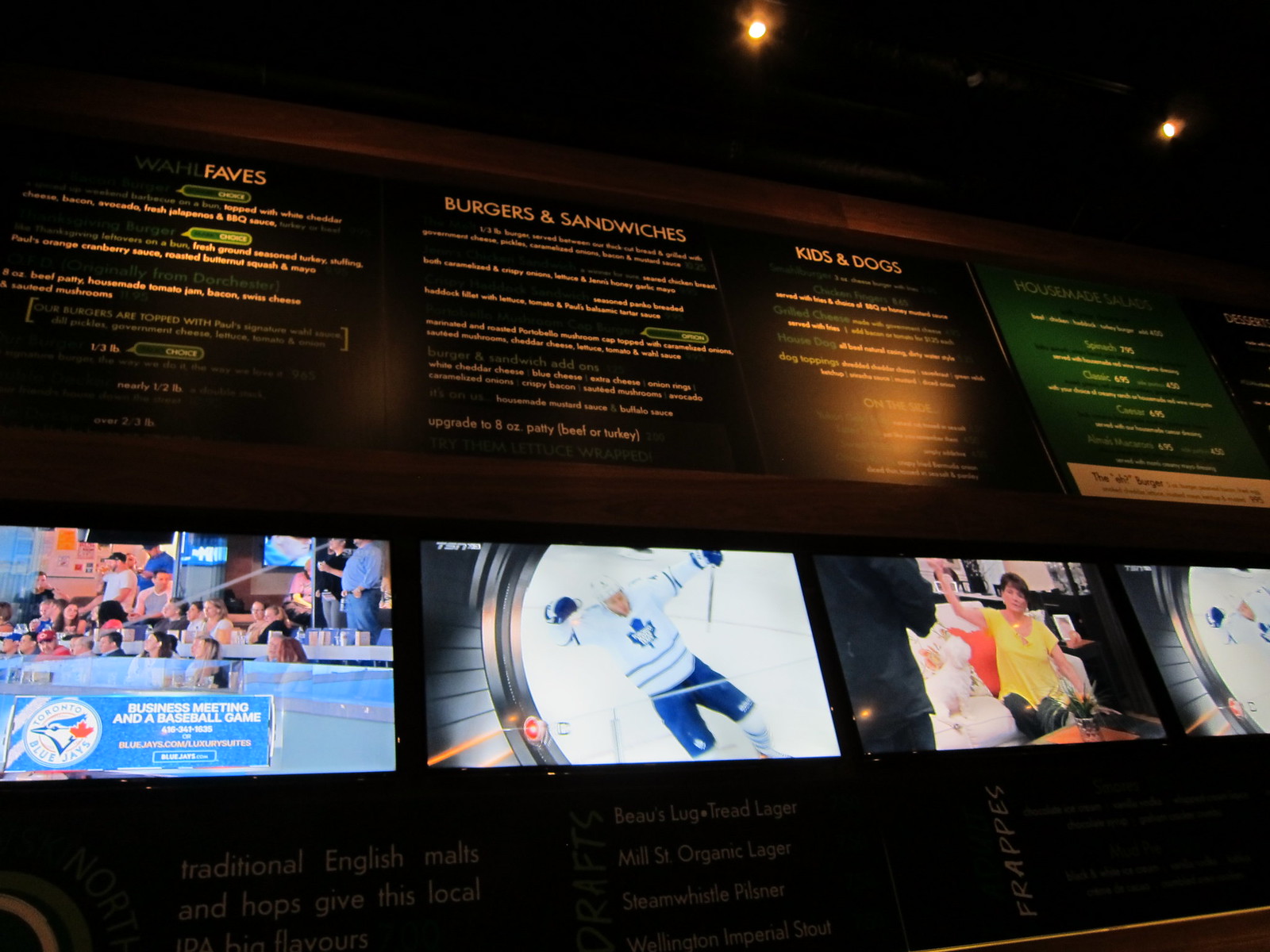The image depicts a wall-mounted menu with a predominantly dark background, featuring bursts of light in certain areas such as the corner and middle sections. The central portion showcases vibrant orange text highlighting various food categories. The menu is divided into several panels, each containing different sections: "Wahl Faves", "Burgers and Sandwiches", and "Kids and Dogs". The rightmost panel has a green background and mentions something related to salads, although the exact text is unclear. Between the top and bottom portions of the menu, there are four color photographs depicting different sports scenes, including a person in a blue and white hockey outfit. Additional details at the bottom of the menu include phrases such as "traditional English malts and hops give this local something big flavors" and a list of available drinks categorized under "drafts" and "frappes". The presence of television-like images or pictures of various sports gives the impression that the menu might be part of a sports bar or restaurant.